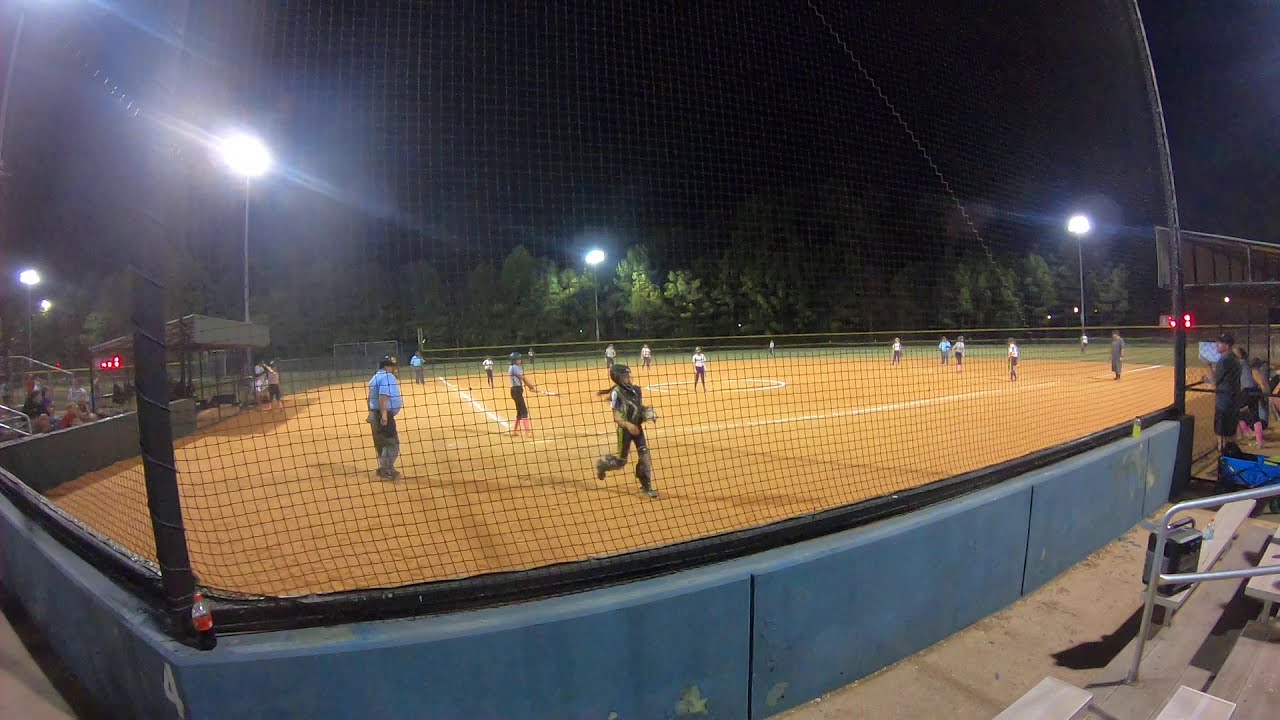The photograph captures a competitive night-time softball game, likely involving high school or college players, taken from the stands behind home plate. The central focus is the softball field illuminated by floodlights, enveloped in darkness, with visible trees in the distant background. At the forefront, a catcher with a ponytail and black-and-yellow gear is running toward the netting, suggesting she is retrieving a foul ball. The umpire, clad in a blue shirt and gray pants, stands behind home plate, alongside a batter dressed in a gray shirt, black pants, and pink cleats, who is poised in the batter's box. Flanking the field are coaches on both the first and third base sides, and a manager with bench players on the far right. The field's layout includes red clay in the infield and grassy outfield areas, populated by around a dozen players in white jerseys and black pants. Spectators occupy the stadium seating, which features a steel handguard, blue low wall, and concrete flooring, partially visible at the bottom right of the image. The scene epitomizes a nocturnal athletic contest, with onlookers scattered in the stands, engrossed in the unfolding game.